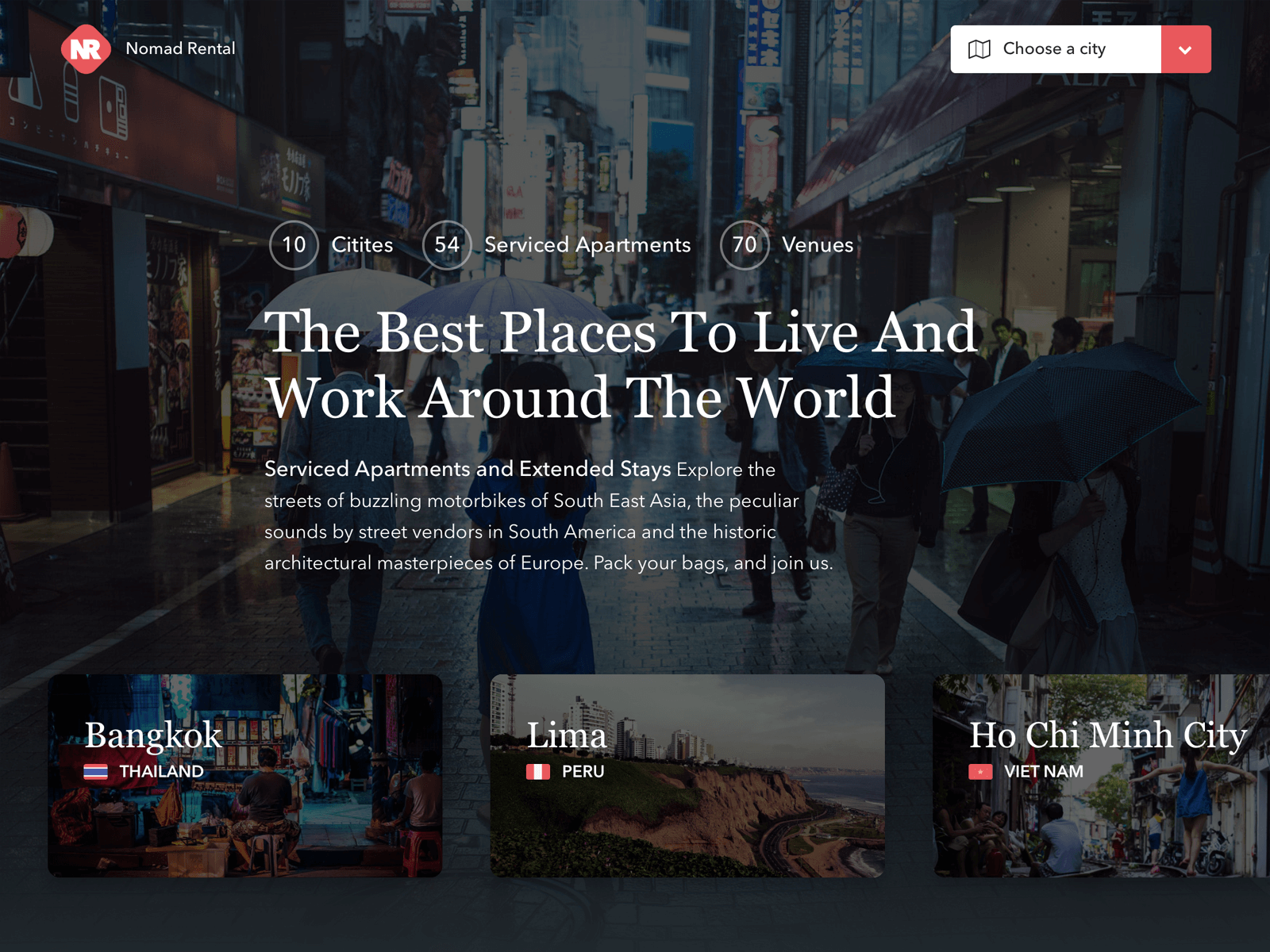Screenshot of a website banner for Nomad Rental

**Top Left Corner:** A red diamond shape with "NR" inside, next to the white text "Nomad Rental."

**Top Right Corner:** A white search box prompting "Choose a City" with a red, pressable button featuring a drop-down arrow.

**Center:** In bold white font, it reads:
"Ten Cities, 54 Service Departments, 70 Venues, Best Places to Live and Work Around the World, Service Departments, and Extended Stays. Explore the streets of bustling motorbikes of Southeast Asia, the peculiar sounds of the street vendors in South America, and the historic architectural masterpieces of Europe. Pack your bags and join us."

**Below Center:** Three thumbnail images labeled:
1. "Bangkok, Thailand" with the Thai flag.
2. "Lima, Peru" with the Peruvian flag.
3. "Ho Chi Minh City, Vietnam" with the Vietnamese flag.

**Background:** A rainy day cityscape scene, showcasing people walking with variously colored umbrellas in blue, white, and purple, creating a charming and aesthetic atmosphere despite the rain.